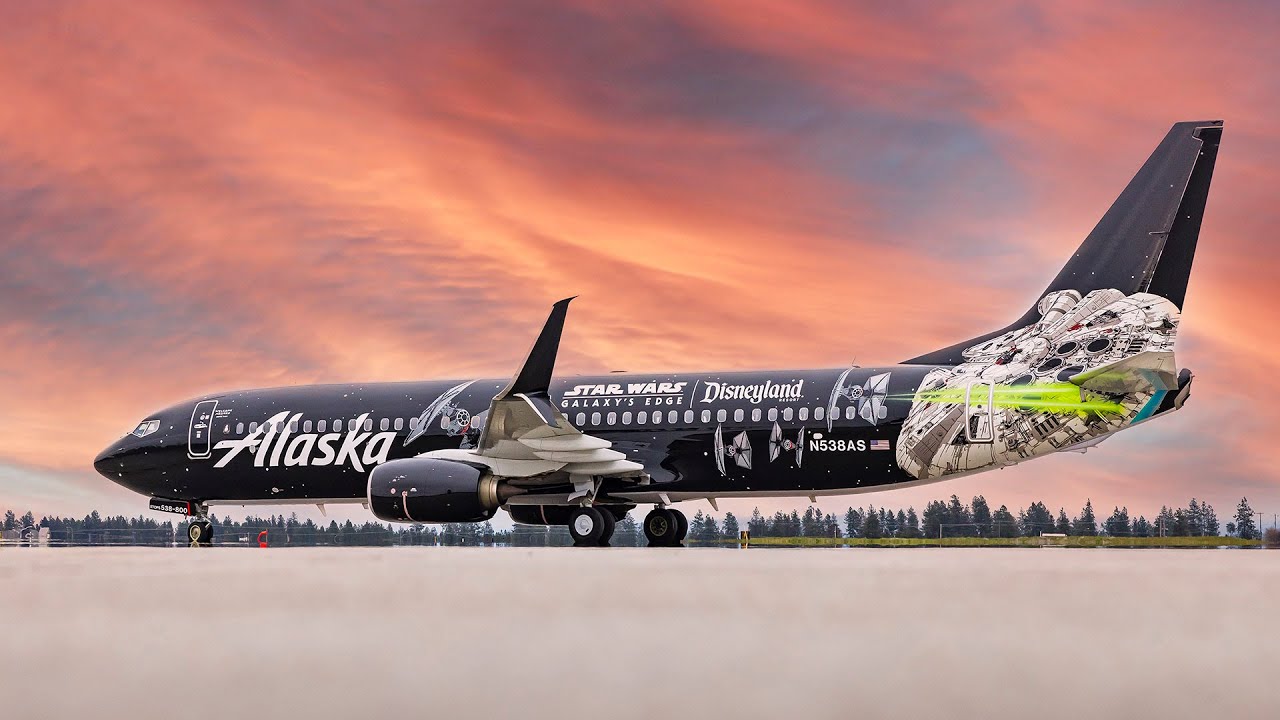This stunning photograph features an Alaska Airlines jet, distinctively decorated to promote Star Wars: Galaxy's Edge at Disneyland. The black airplane is prominently adorned with white lettering that reads "Alaska," "Disneyland," and "Star Wars Galaxy's Edge." A closer look reveals detailed artwork, including a dramatic depiction of TIE fighters engaging in a battle with the Millennium Falcon on the plane's tail, complete with vivid pew, pew, pew laser blasts. The jet, identifiable by the registration number N538AS and an adjacent U.S. flag, appears to be a Boeing model, recognized by its twin engines and sizable fuselage with over 30 windows, suggesting ample passenger capacity. The backdrop of the image is equally breathtaking, with a vibrant sunset painting the sky in shades of red, orange, pink, and blue, featuring a tree line of evergreens. The airplane, positioned in the middle third of the frame, angles away to the left as it rests on the runway, set against the enchanting twilight sky.